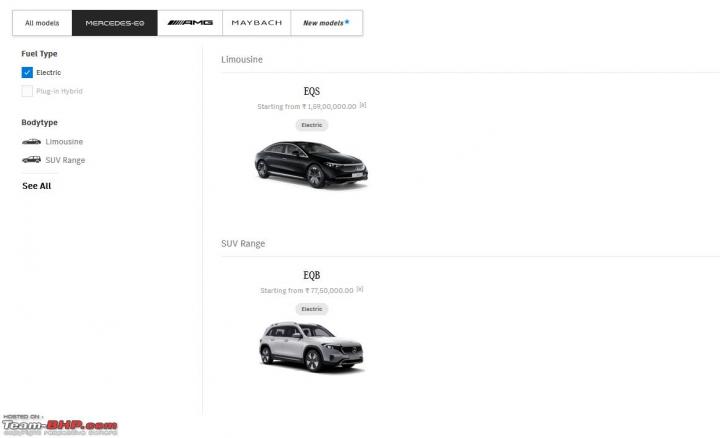This image features a clean, white background showcasing a series of car listings for Mercedes-Benz models. At the top, it displays headings such as "All Models," "Mercedes E-Zero," "AMG," and "Maybach," indicating the variety of vehicles being offered. 

Detailed text segments highlight key attributes of the available models, focusing on new electric offerings and their specifications. Under "Fuel Type," it specifies "Electric," while "Body Type" categorizes the vehicles as "Limousine" and "SUV Range."

Specifically, the black Mercedes EQS Limousine is listed with a starting price of 16,900,000, whereas the white Mercedes EQB SUV Range starts from 7,750,000. Various sections on the page provide in-depth details about these luxury electric models, emphasizing their high-end features and attractive starting prices.